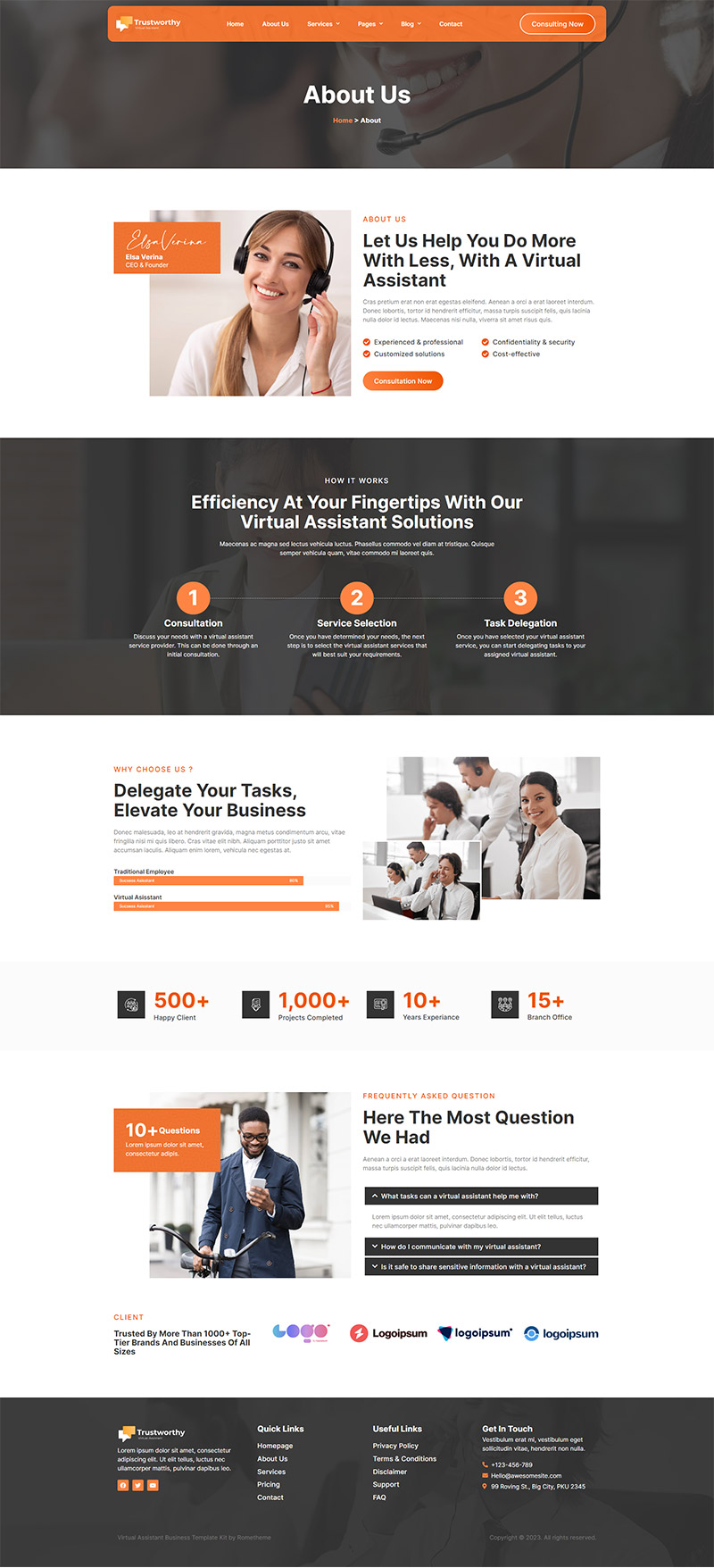**Website Template Screenshot Description:**

This screenshot showcases a template website designed for desktop viewing, characterized by a sleek color scheme of various shades of gray complemented by vibrant orange accents. 

At the top of the page, an orange header features a menu bar, with the "About Us" section currently selected. Below the header, there's a large, grayed-out background image of a woman smiling and talking into a microphone.

The central part of the page features a professional-looking woman with long blonde hair tied in a ponytail, wearing a headset. This full-face and chest shot is set against an orange field displaying her signature. To the right of this image, a text section reads, "Let us help you with [...] the virtual assistant," followed by various service options.

Directly below, a gray banner highlights the phrase "Sufficient to use fingertips with a virtual assistant," accompanied by three numbered orange circles labeled "Consultation," "Service Selection," and "Task Delegation."

Further down, imagery includes a group of people in white business suits, all wearing headsets, with the tagline "Delegate your tasks, elevate your business" positioned alongside orange and gray bars showcasing statistics: over 500 happy clients, 1,000 projects completed, and 10 years of experience.

The page also displays an image of a man in a long coat pushing a bicycle while smiling and looking at his phone. This section highlights "10+ most asked questions," although the accompanying text is too small to read.

Towards the bottom, various logos are displayed, followed by a footer containing the business address and additional contact information.